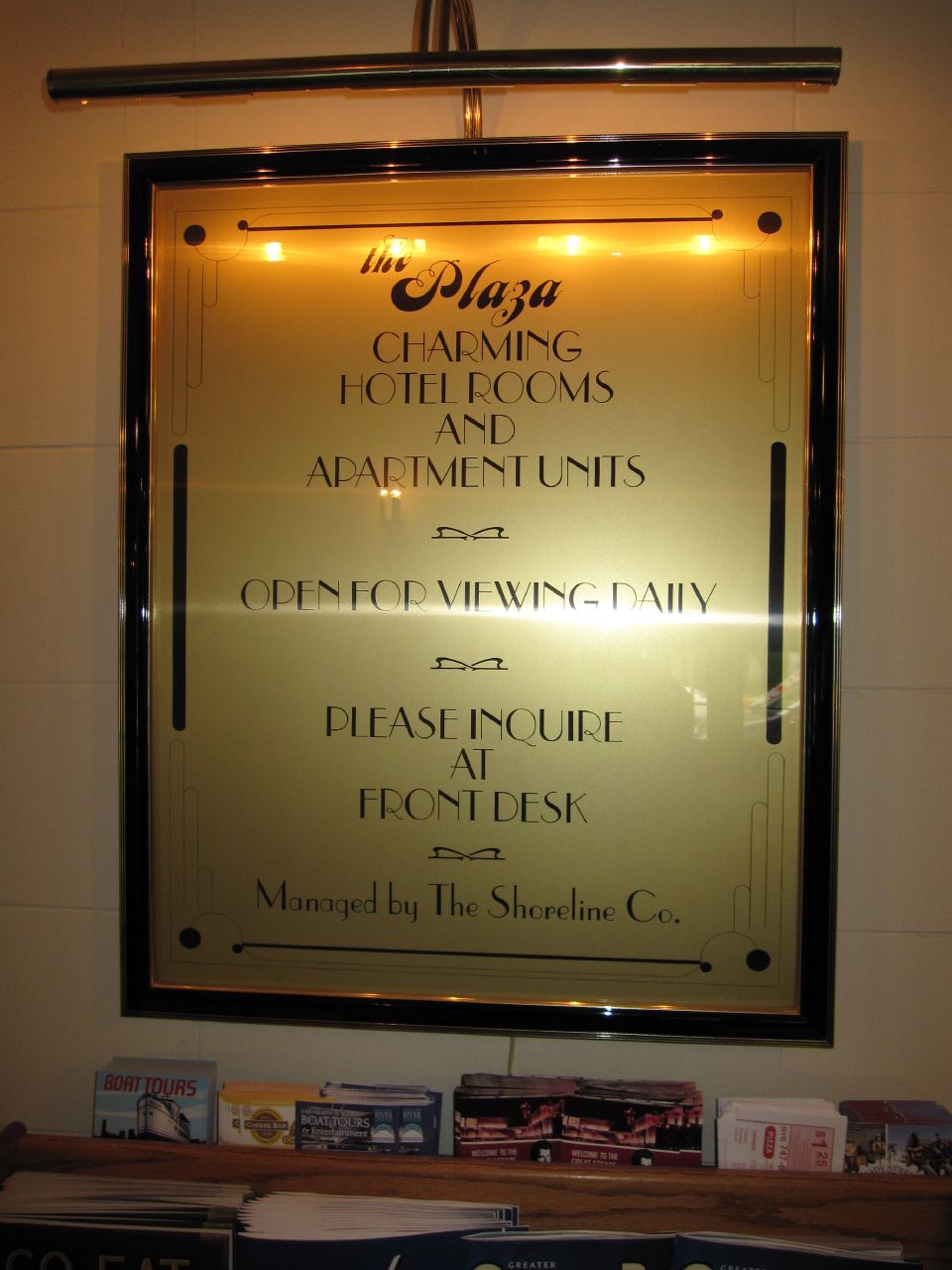The image showcases an indoor scene featuring a centrally-hung plaque framed in dark lacquer. The gold-lettered sign reads, "The Plaza, Charming Hotel Rooms and Apartments. Open for viewing daily. Please inquire at front desk.” Lower in smaller text, it mentions, "Managed by the Shoreline Company." A light fixture is mounted above the sign, illuminating it. Beneath the plaque, a wooden display case holds several pamphlets about boat tours and various attractions, along with an open three-ring binder and some coupons. The setting is inside a hotel, as indicated by the neatly organized information for guests. The scene is enriched with a palette of colors including white, gold, yellow, orange, tan, blue, red, purple, pink, brown, and black.